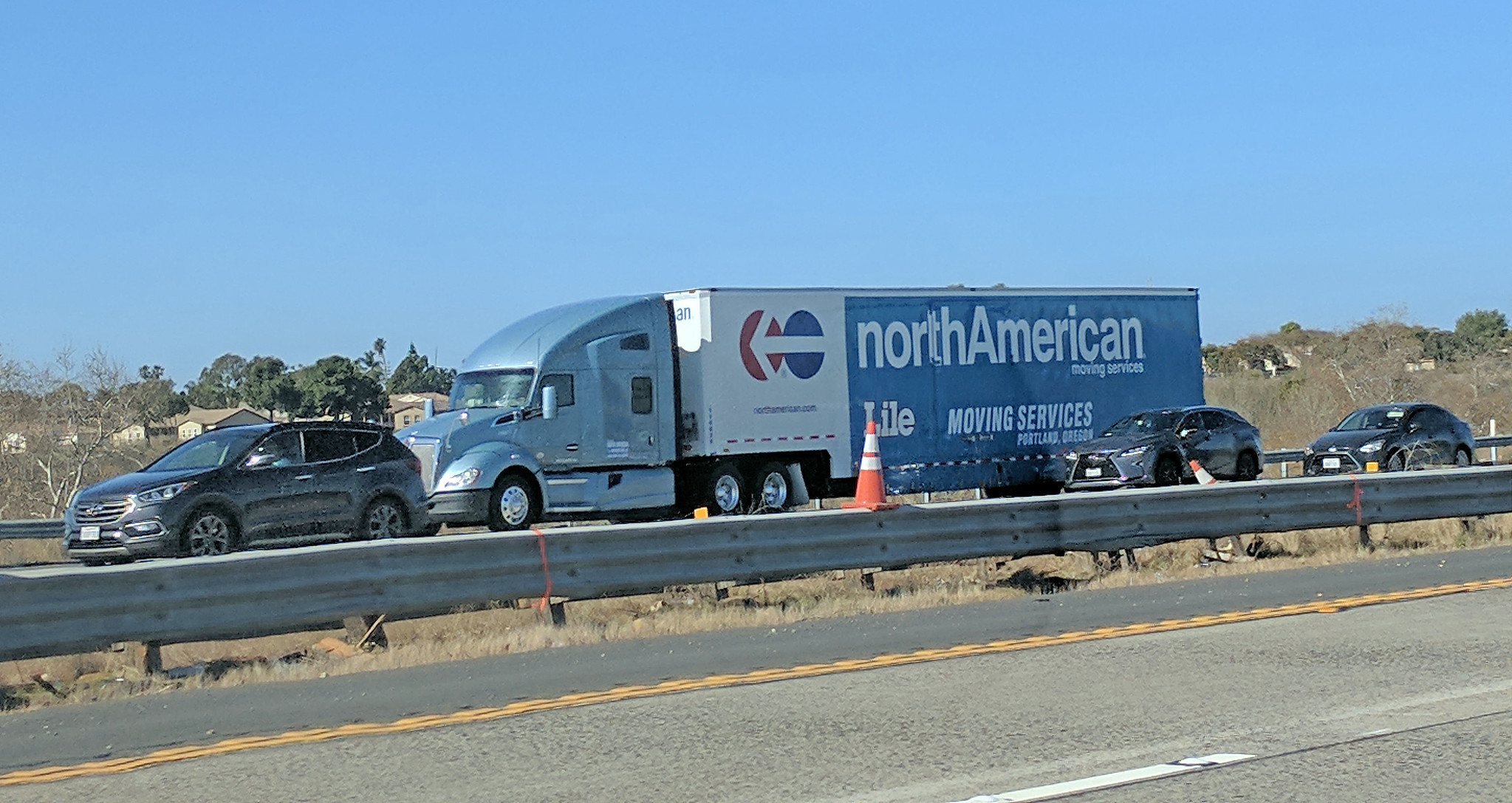The photograph captures a busy highway scene taken from one lane, offering a comprehensive view of the adjacent lane separated by a metal guardrail. An orange traffic cone with two white stripes is perched atop this guardrail. On the opposite lane, there are three cars and a semi-truck arranged in a staggered formation. The two cars trail behind the semi-truck, which occupies the middle position, while another car leads at the front. The cars are all varying shades of silver-gray to dark gray and have tinted windows. The semi-truck is notably large and blue, featuring black tires and a distinctive trailer emblazoned with "North American Moving Services," accompanied by an arrow pointing forward. In the background, a few arid desert hills with sparse trees can be seen, along with a residential neighborhood to the left. The sky is a clear, vivid blue with no clouds in sight.